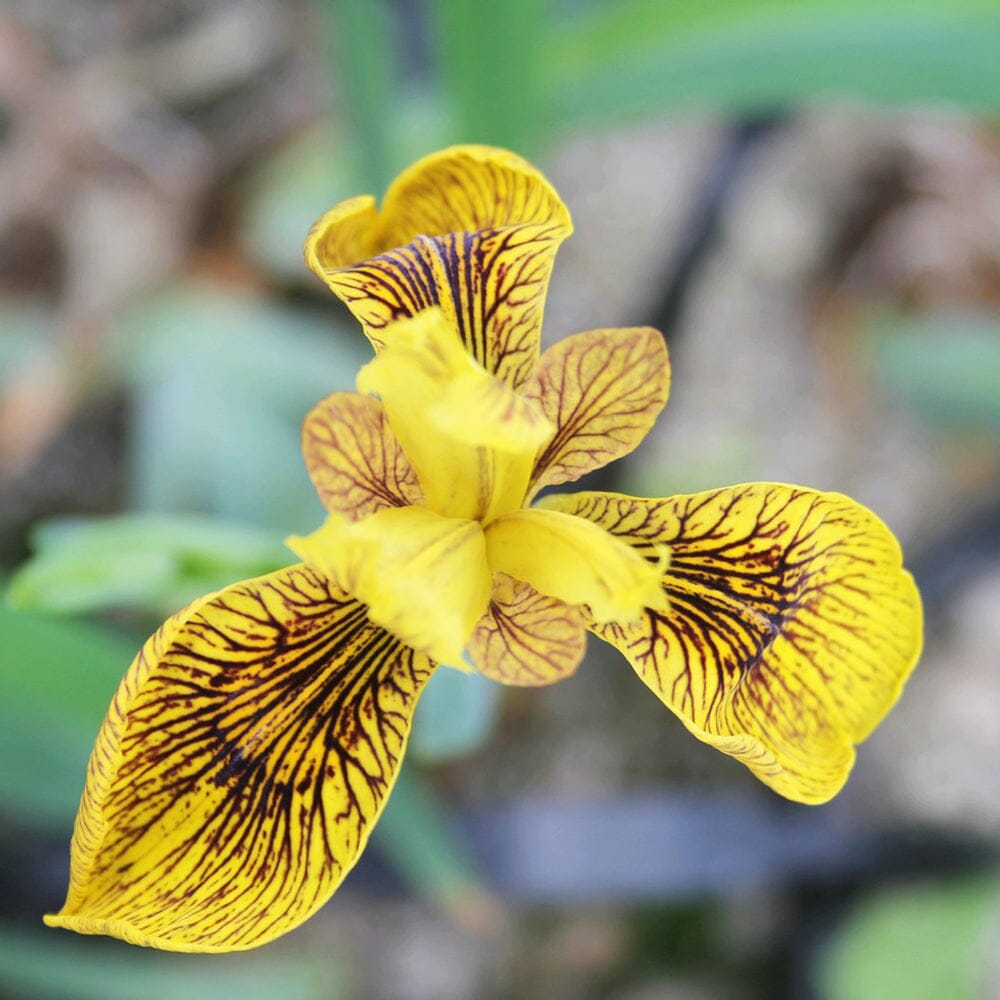This outdoor daytime photograph features a close-up view of a striking yellow flower at the center, with a blurred background of green leaves and brownish elements. The square-shaped image measures approximately six inches by six inches. Dominating the flower are three large, shiny yellow petals adorned with prominent, thick brown veins, each petal positioned with one extending upwards and the other two extending towards the lower left and lower right. Nestled between these large petals are three smaller yellow petals showcasing the same brown veining, though the veins are less pronounced. From the flower's center, three additional bright yellow petals emerge, standing upright and decorated with subtle, light brown vertical veins that do not extend to the edges. The overall focus on the flower contrasts beautifully with the soft, blurred green and brown hues in the background, highlighting the intricate details of the petals and their vein patterns.